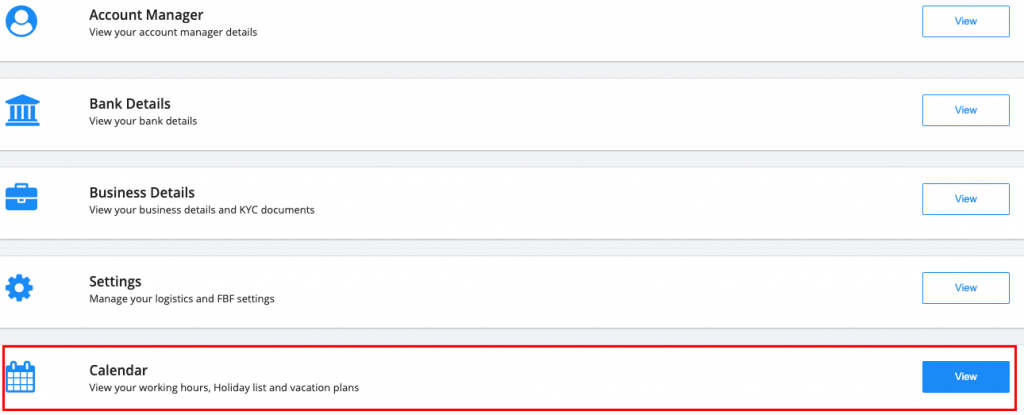This image showcases a sophisticated business management application interface, designed with a landscape orientation and predominantly white background. The interface features blue accent colors, utilized for icons and buttons throughout the application. These buttons are color-coded: white inside when not selected and blue inside when selected, providing a clear visual cue for user interactions. 

Each section is distinguished by long horizontal banners separated by gray gutters, each banner paired with a relevant and simply-styled icon. Here are the sections detailed from top to bottom: 

1. **Account Manager**: Allows users to view account manager details.
2. **Bank Details**: Provides access to view bank details.
3. **Business Details**: Enables users to view business details and KYC documents.
4. **Settings**: Lets users manage logistics and FBF settings.
5. **Calendar**: Allows users to view working hours, holiday lists, and vacation plans. 

Notably, the Calendar section features a dark blue button for viewing, highlighted by a red box, indicating this might be a focal point in a presentation explaining the functionality of each element. This presentation-like setup suggests an instructional or demonstrative context, but the exact type of application and platform remain unspecified due to the cropped nature of the screenshot. This cropped view exclusively shows the described banners without revealing additional contextual information about the application.